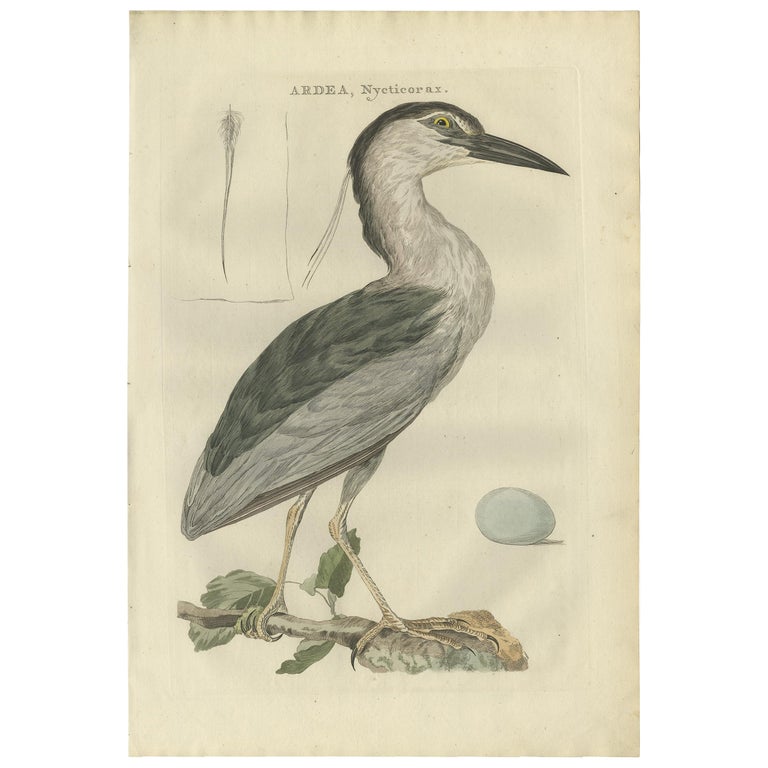This detailed illustration depicts a large bird, likely a heron or an egret, with very long legs standing gracefully on a tree limb adorned with a few small leaves. The artwork is rendered in black and white on a beige background, resembling a hand-drawn sketch. The bird presents a striking color palette: its sharp, black beak contrasts sharply with the white feathers covering its neck, face, and chest, while the top of its head, back of the neck, and wings are shaded in black and dark gray. Intricate details include a light gray area around its etched eye, yellow feet with black nails, and three tendril-like appendages extending from the back of its head. Positioned in front of the bird is a light blue egg, adding a touch of color to the otherwise monochromatic scene. Above the bird, the text "Ardea nycticorax" suggests its scientific name.